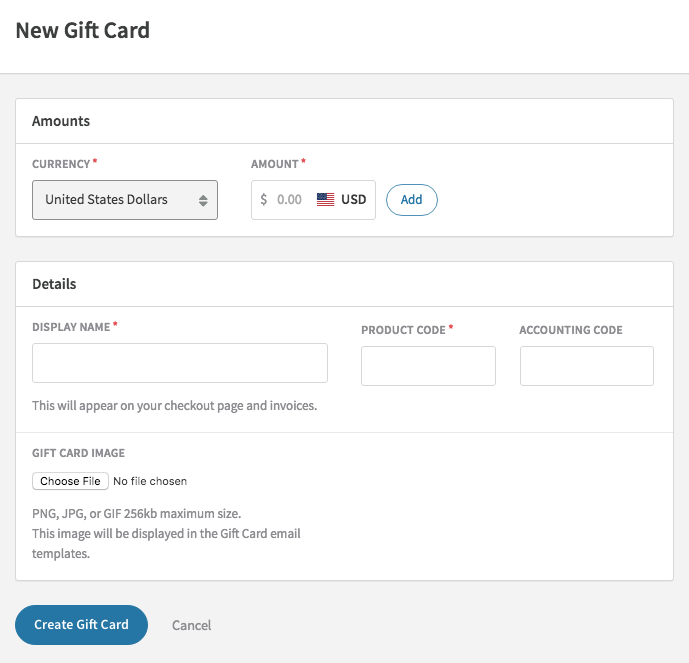This image is a detailed screenshot of a user interface for creating a new gift card. In the upper left-hand corner, there is a heading labeled "New Gift Card." Directly beneath this, it specifies that the amounts and currency are set to United States Dollars (USD), and the current amount is listed as zero. An option to add an amount appears once a value has been input. Below these details, there is a section titled "Details," which includes input fields for various pieces of information such as Display Name, Product Code, and Accounting Code, with the note that these will appear on checkout pages and invoices. Further down, users are prompted to select a Gift Card Image by choosing a file. Accepted file formats are PNG, JPG, or GIF with a maximum file size of 256KB, and it notes that this image will be featured in the gift card email template. Finally, in the lower left-hand corner, there are two options to either Create Gift Card or Cancel.